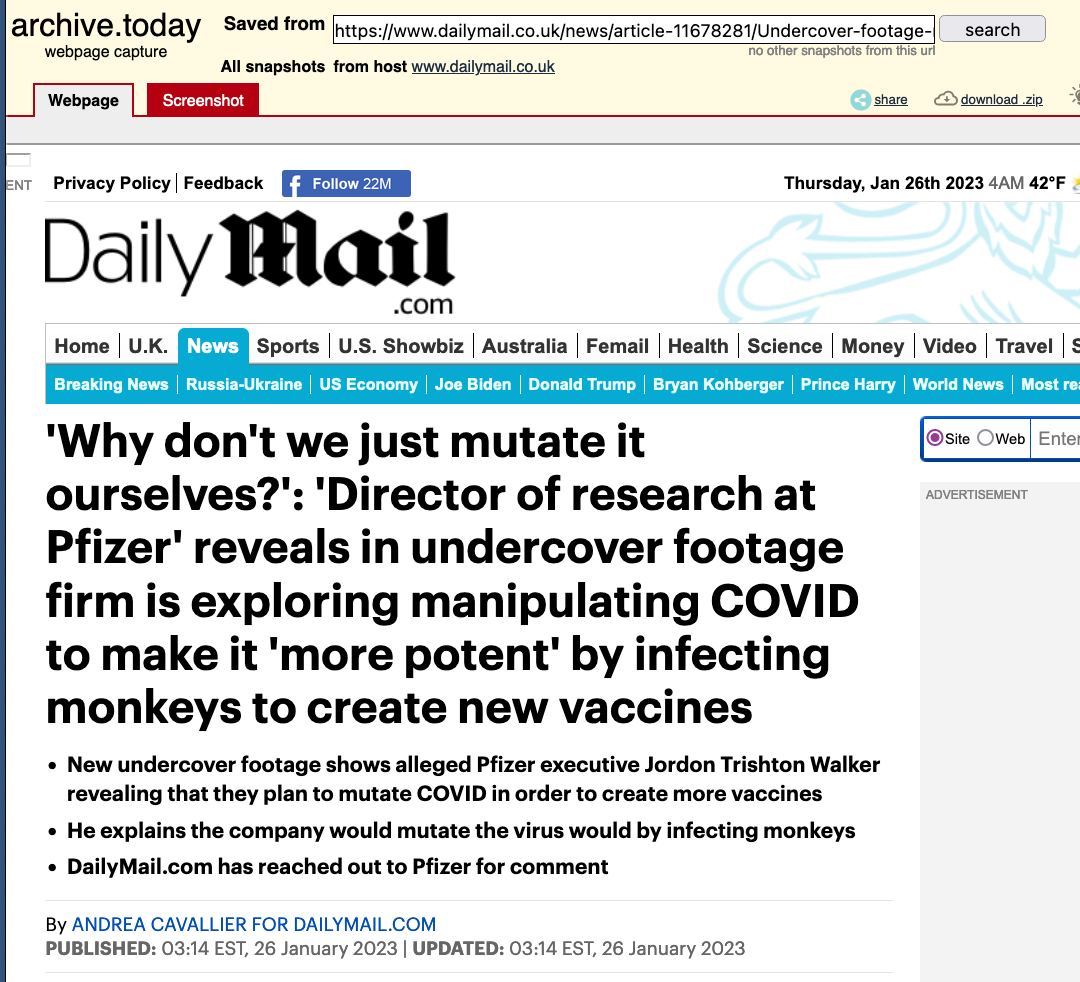The image displays a screenshot of a webpage captured on the archive.today website. At the top, there is a light yellow banner with text that reads "archive.today". Below this banner, there is a section labeled "Webpage Capture" followed by a "save from URL" field and a search function indicated by a grey box. Further down, you see the text "All snapshots from host www.dailymail.co.uk" indicating that this capture is from the Daily Mail website.

Moving down, a grey banner contains the text "Webpage" on the left, and a red box with white text that says "screenshot" on the right. Below this grey banner, the image displays a white background with small print that includes "Privacy Policy" and "Feedback". There is also a noteworthy blue rectangle with an option enticing visitors to "Follow 22 Million on Facebook."

Displayed prominently is the date and time: "Thursday, January 26, 2023, 4am" along with the current temperature of "42 degrees Fahrenheit". The website heading showcases "dailymail.com," with sections such as "home," "UK," and a highlighted "news" tab in blue.

Further down, under the "breaking news" section, there are topical categories listed: "Russia," "Ukraine," "U.S. economy," "Joe Biden," "Donald Trump," "Brian Kohlberger," "Prince Harry," "world news," and "most read."

The white background at the top indicates additional sections: "sports," "U.S.," "showbiz," "Australia," "Femail (stylized as F-E-M-A-I-L)," "health," "science," "money," "video," and "travel."

Finally, a heading introduces various bullet points that elucidate different news items, making it clear that the page is rich with diverse news content.